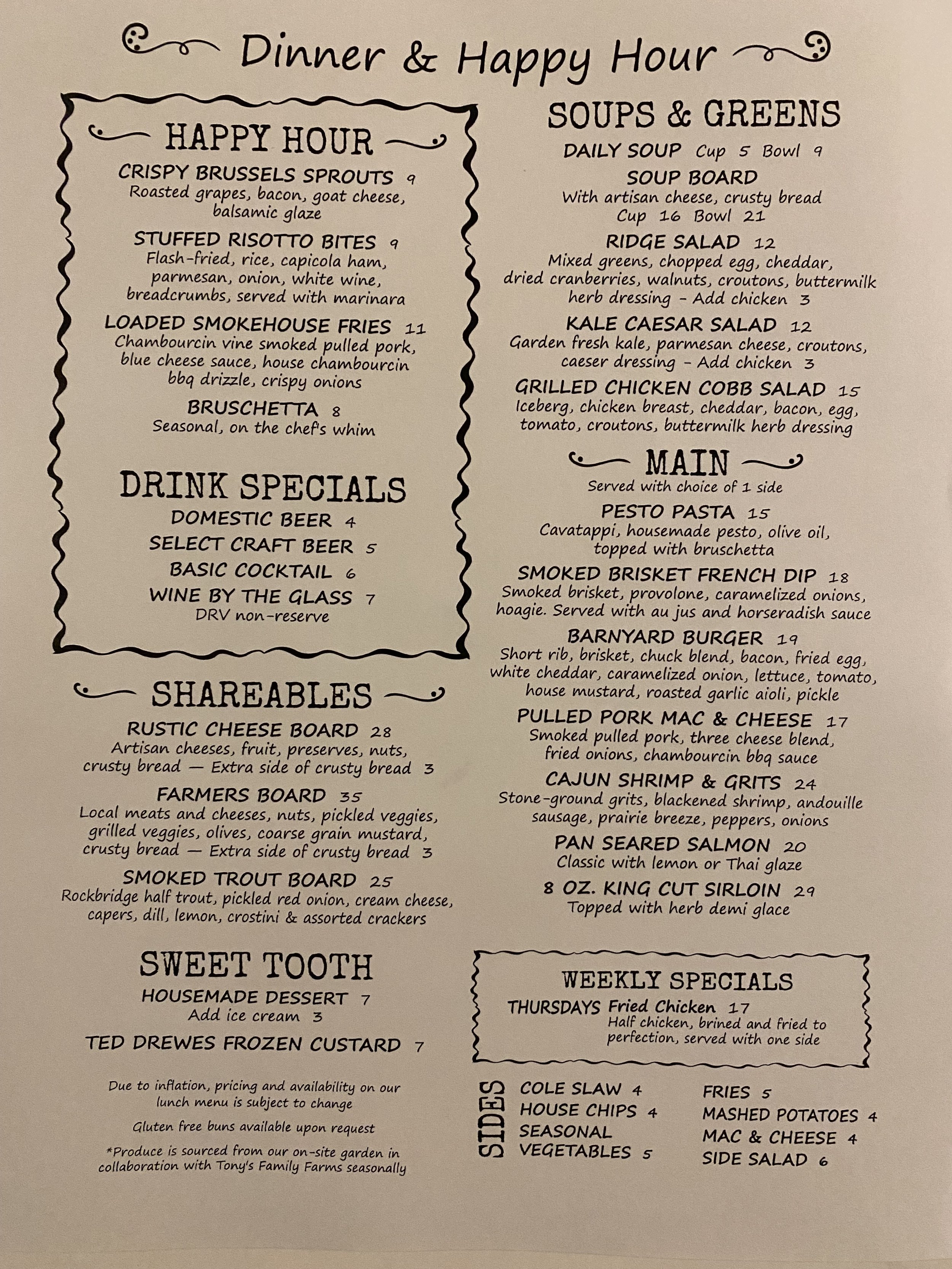The vertical, rectangular image showcases a black and white restaurant menu printed on light brown paper. The menu is titled "Dinner and Happy Hour" and features sections outlined with black squiggly lines. The Happy Hour section lists specials like crispy Brussels sprouts with roasted grapes, bacon, goat cheese, and balsamic glaze for $9, as well as stuffed risotto bites for $9. Drink specials include domestic beers for $4, select craft beers for $5, basic cocktails for $6, and wine by the glass for $7. The Shareables section offers various boards such as the rustic cheese board for $28. The Sweet Tooth section highlights homemade desserts for $7, with an option to add ice cream for an additional $3. Other sections include Soups and Greens with items like daily soup and grilled chicken cobb salad, and the Main menu featuring dishes like smoked brisket French dip, Cajun shrimp and grits, and an 8 oz King Cut Sirloin. A boxed area at the bottom right lists the weekly specials, including Thursday's special: fried chicken. Prices are displayed in round numbers throughout the menu.